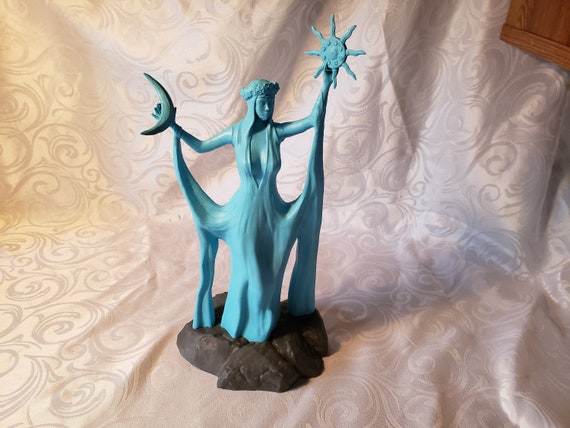The image depicts a turquoise-colored clay statue of a mystical goddess, adorned with a crown of flowers around her head and standing on a brown rocky base. The goddess is clothed in a long, halter-style robe that is attached to her wrists, causing the lower sides of the dress to lift when her arms are outstretched. Her exposed chest is modestly covered by the robe. In her left hand, she holds an eight-pointed star-like symbol with a circular structure and dots inside, while her right hand raises a crescent moon. The statue sits on a velvety, pink cloth with swirl patterns that drapes over an unseen surface, enhancing the ethereal quality of the scene.